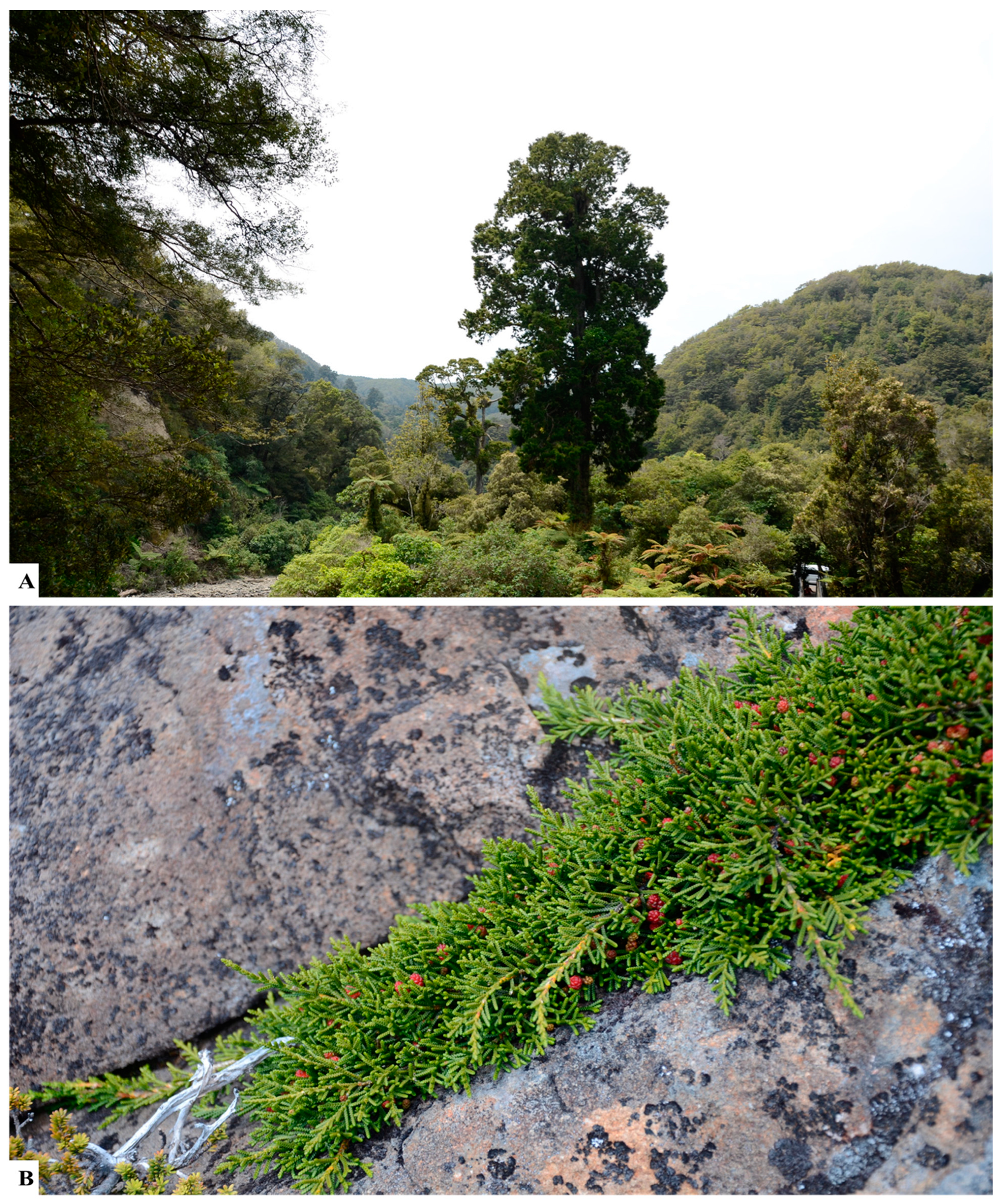Here are two related outdoor photos labeled A and B. In the top photo (A), a tall tree stands prominently amidst a diverse array of trees and bushes, creating a rich tapestry of greens. The scene depicts a forest that is bathed in natural daylight, showcasing various shades of light green, dark green, and light orange or light blue. In the bottom photo (B), the rocky ground is featured with a unique setup of stones interspersed with moss or ferns. A tree adorned with red berries is visible, along with some white string intricately draped over the rocks and bushes. The brown earth contrasts with the vibrant foliage, enhancing the depth and detail of the scene. Both photographs capture the essence of the forest with their daytime lighting and natural beauty.